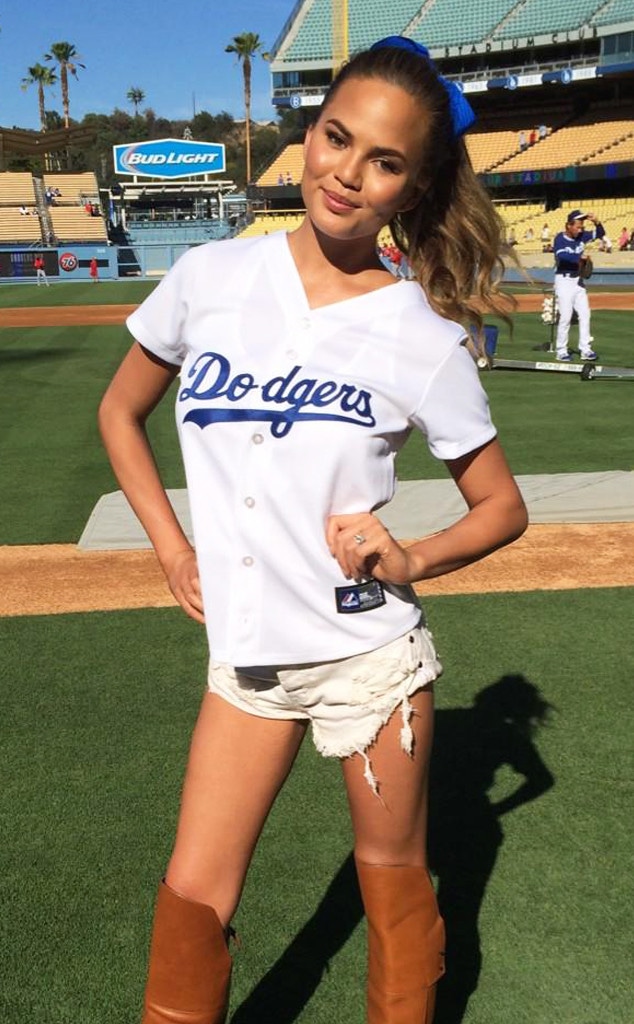In the image, Chrissy Teigen is posing confidently in an empty baseball stadium, likely the LA Dodgers' field. She's wearing a distinctive white Dodgers baseball jersey with "Dodgers" emblazoned in blue cursive on the chest. Her ensemble is completed with short white shorts that are frayed at the bottom and knee-high camel-colored boots. A blue ribbon adorns her hair, tied back in a ponytail. Chrissy stands with her hands on her hips, giving a slight smirk to the camera. The vivid green of the baseball field stretches out behind her, with a baseball player in a Dodgers uniform visible to the right. The backdrop includes empty multi-tiered seating and a prominent Bud Light sign to the left. Further in the distance, you can spot tall palm trees under a clear blue sky.